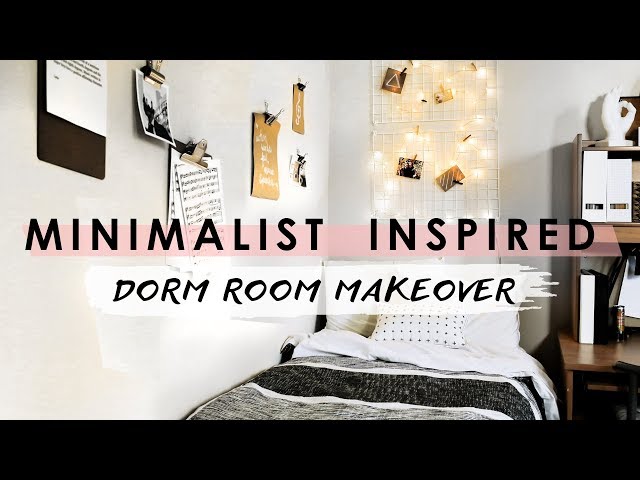The image titled "Minimalist Inspired Dorm Room Makeover" is presented with black letterbox borders at the top and bottom, suggesting it might be a screenshot from a YouTube video or a magazine page. In the foreground, the title text in uppercase black letters is displayed, accented by a pink underline. The background reveals a well-organized dorm room, specifically the sleeping area.

The room features a twin bed adorned with a patterned bedspread in shades of black, white, and gray, and a pillow with black dots on a white background. Behind the bed is a stylish checkerboard design adorned with various pictures attached using clothespins, softly illuminated by a string of lights. To the left of the bed, the white walls are decorated with clipboards holding sheets of music, phrases, and other notes, creating a functional yet aesthetic display.

To the right of the bed is a brown desk cluttered with books, folders, and files. Atop the desk sits a delicate resin OK symbol hand. This minimalist-inspired setup perfectly blends practicality with modern design, offering both comfort and style in a compact dorm room setting.